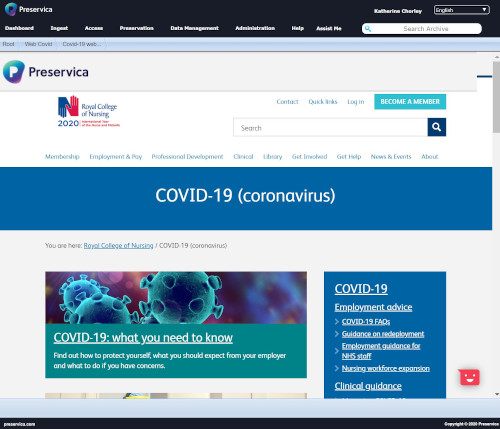The image captures a webpage from the Royal College of Nursing, prominently displaying the Preservica logo at the top, framed by a black border. To the top-left, the name "Catherine Chesney" is displayed, with the word "English" beside it, indicating the language setting. The left sidebar contains navigational links such as "Dashboard" and "Access," alongside other clickable options.

Central to the page is a section dedicated to COVID-19 information. At the top of this section, "COVID-19 (Coronavirus)" is written in large letters on a vibrant blue background. Below this, a white section labeled "COVID-19: What You Need to Know" offers essential information. The background of this section is colorful, featuring a multicolored pattern of pink, orange, green, and blue, accompanied by an image of COVID-19 cells.

Toward the right side, an "N" logo is displayed, half-red and half-blue, with the year "2020" beneath it. Below this, there are quick links labeled "Contact," "Quick Links," "Login," and "Become a Member," with "Become a Member" highlighted in teal.

Further down the page, there is a search bar accompanied by a question icon. Below this are various sections labeled "Membership," "Employment," "Professional Development," "Checkout," "Library," "Get Help," "Experts," and "About." Featured prominently on the page is a blue box with "COVID-19" written inside, offering employment advice, guidance for staff, and links to COVID-19 FAQs.